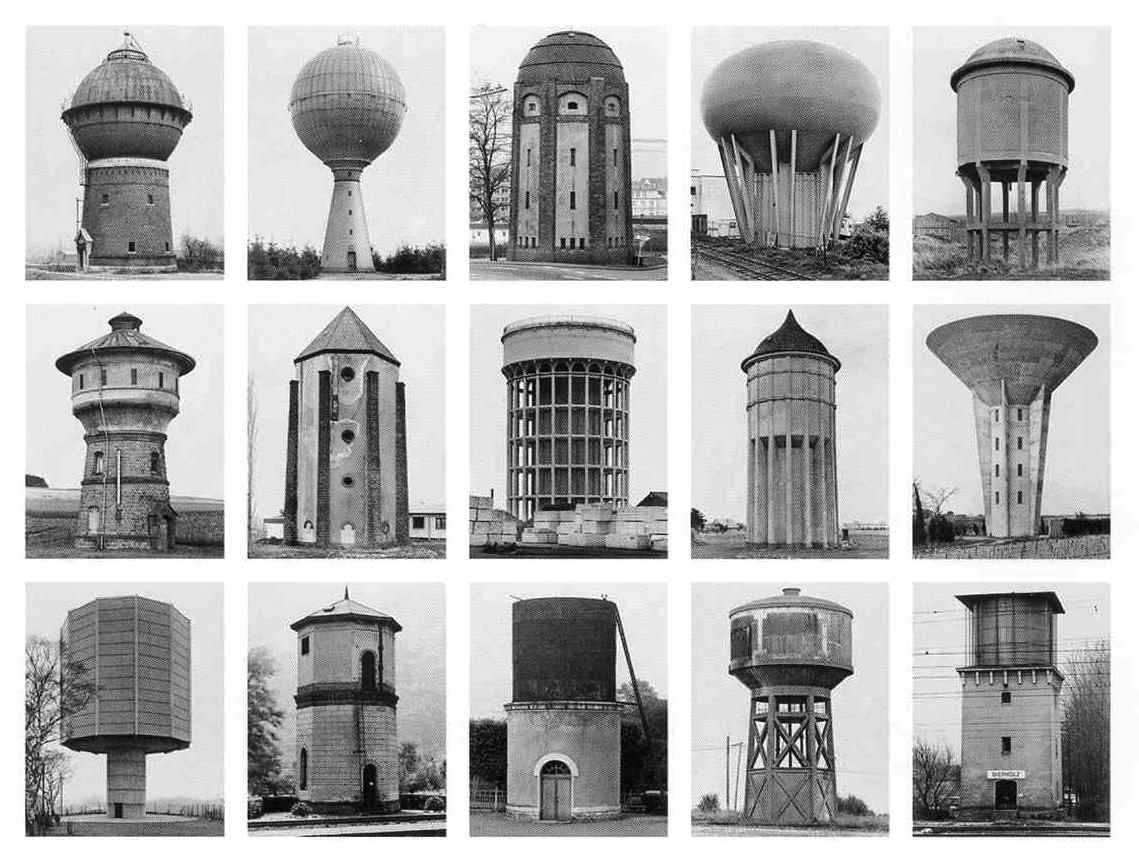This black and white image features a grid of 15 smaller rectangular photographs, each depicting a distinct type of tower structure, arranged in a 5-by-3 layout with white spaces separating them. The towers showcased span various architectural styles and eras, highlighting their evolution over time. Dominantly, these structures appear to be water towers, exhibiting a range of designs from dome-shaped tops, reminiscent of modern water storage solutions, to more intricate, Victorian-style towers with pointed rooftops and elaborate details. Some towers are cylindrical with conical roofs, while others feature combinations of shapes such as a thin circular base supporting a larger circular top, or square bases transitioning into different forms. The imagery captures not only the structural diversity but also the textures unique to these historical edifices, evoking a sense of architectural progression.